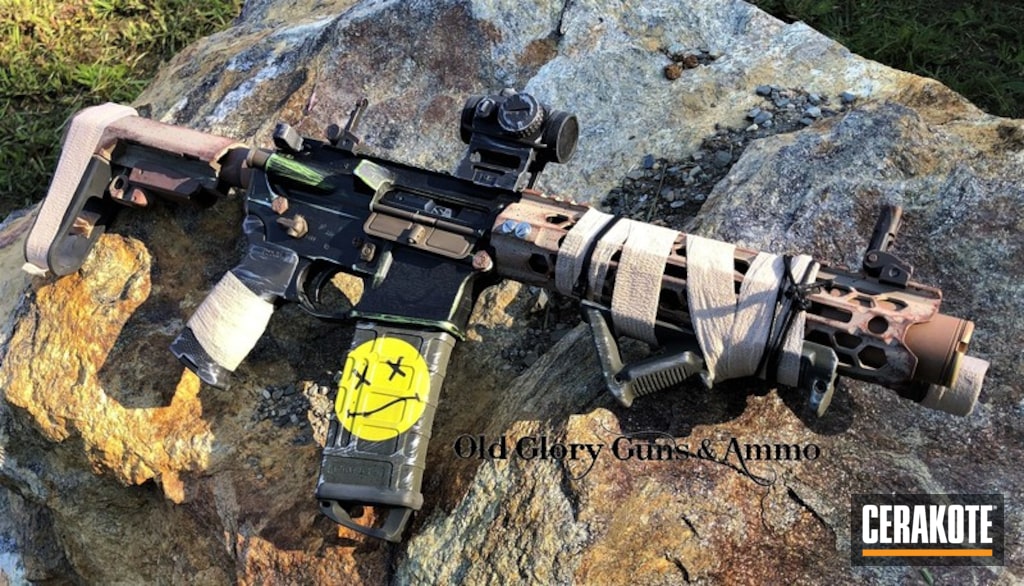The photograph captures a large black rifle, prominently displayed against a giant, gray boulder in an outdoor setting. The rifle, angled with the front end pointing to the bottom right and the stock to the top left, features a black scope mounted on top. Wrapped around the rifle's barrel and body is a bandage-like white tape, presumably for added comfort while holding. Distinctively, the rifle's magazine cartridge displays a sticker of a yellow face with X-shaped eyes and a frowning, squiggly mouth, suggesting a grim expression. In a black see-through box with white letters at the bottom right-hand corner of the image is the brand name "Cerakote," underlined by a yellow line. Directly beneath the rifle, the text "Old Glory, Guns and Ammo" is clearly visible.